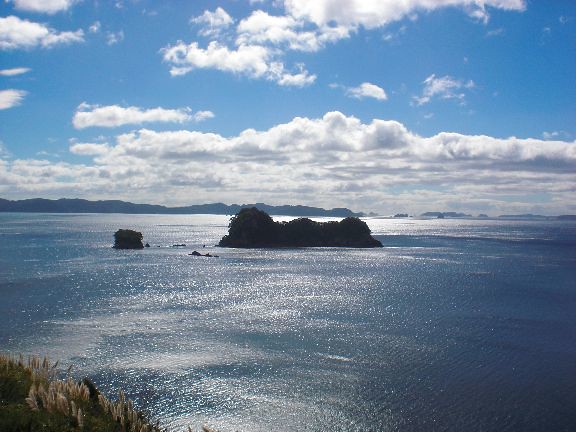The image is a square photograph capturing a tranquil outdoor scene by the water's edge. The lower part of the image, extending up to the middle, features a calm stretch of blue-gray water with some white reflections glinting where sunlight hits the surface. In the foreground, the bottom left corner reveals a patch of tall grass. Near the center of the water, there is a small island adorned with vegetation, characterized by three peaks—one larger peak on the left and two smaller ones to the right. To the left of this island rests a prominent stone. In the distant background, a rocky, hilly landscape outlines the horizon, merging seamlessly with the serene expanse of water. Above, the upper half of the picture showcases a bright blue sky filled with patches of white, puffy clouds with gray undersides, contributing to the image's peaceful ambiance. The overall scene is one of tranquility, with a mixture of natural elements—from the grassy foreground and peaceful water to the distant hills and cloud-strewn sky.